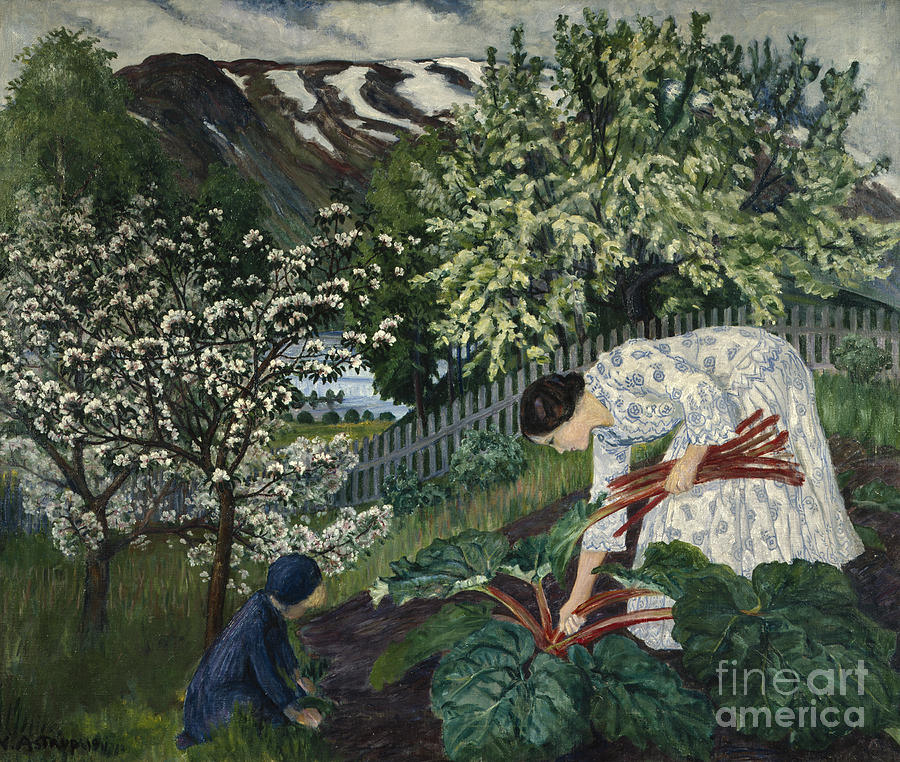This detailed painting titled "Fine Art America" in the bottom right corner captures a serene garden scene featuring a woman and a young girl engaging in gardening activities. The woman, adorned in a white and light blue gown with floral patterns, bends down to pick rhubarb or large-leafed vegetables. She has dark brown or grey hair. Nearby, the little girl, dressed in a dark blue frock and bonnet, kneels by the edge of the garden, touching the soil but not actively pulling any plants. 

The garden is bordered by a wooden or white picket fence with a wavy pattern, adding a cozy charm to the scene. Surrounding the figures are scattered trees; to the left are trees with white flowers and brown trunks, while the background features taller trees with a mix of dark and light green foliage. The setting is further enriched by a grassy landscape and a gentle river in the distance.

In the upper part of the image, snow-capped mountains rise majestically against a mostly cloudy sky. The unique blend of dark and light blues in the sky suggests either an evening or early morning time. The tranquil atmosphere and fine details reflect the painting's fine arts essence, inviting viewers into a peaceful, pastoral moment.